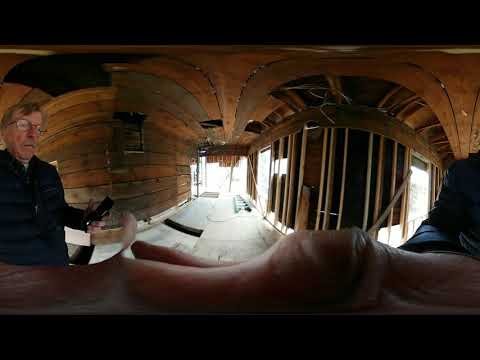This photograph captures the interior of a house under construction, likely of an older building undergoing refurbishment. The scene has been taken as a 360-degree panoramic shot, evidenced by the distortion at the bottom where the photographer's fingers appear warped. The construction site features wooden slats forming portions of the walls and ceiling, with visible gaps and exposed studs indicating incomplete structures. Sunlight streams through blank spaces on the far right and center, likely future windows or doorways. On the left, wooden planks line the wall, while a ladder lies on the floor in the middle of the room. An older gentleman, who appears to be the photographer, is visible in the image. He wears a black jacket, a blue shirt, glasses, and sports a mustache and short gray hair. Holding a phone in his left hand, he appears on the left side of the photograph, with a second image of his left arm appearing on the right due to the panoramic effect.